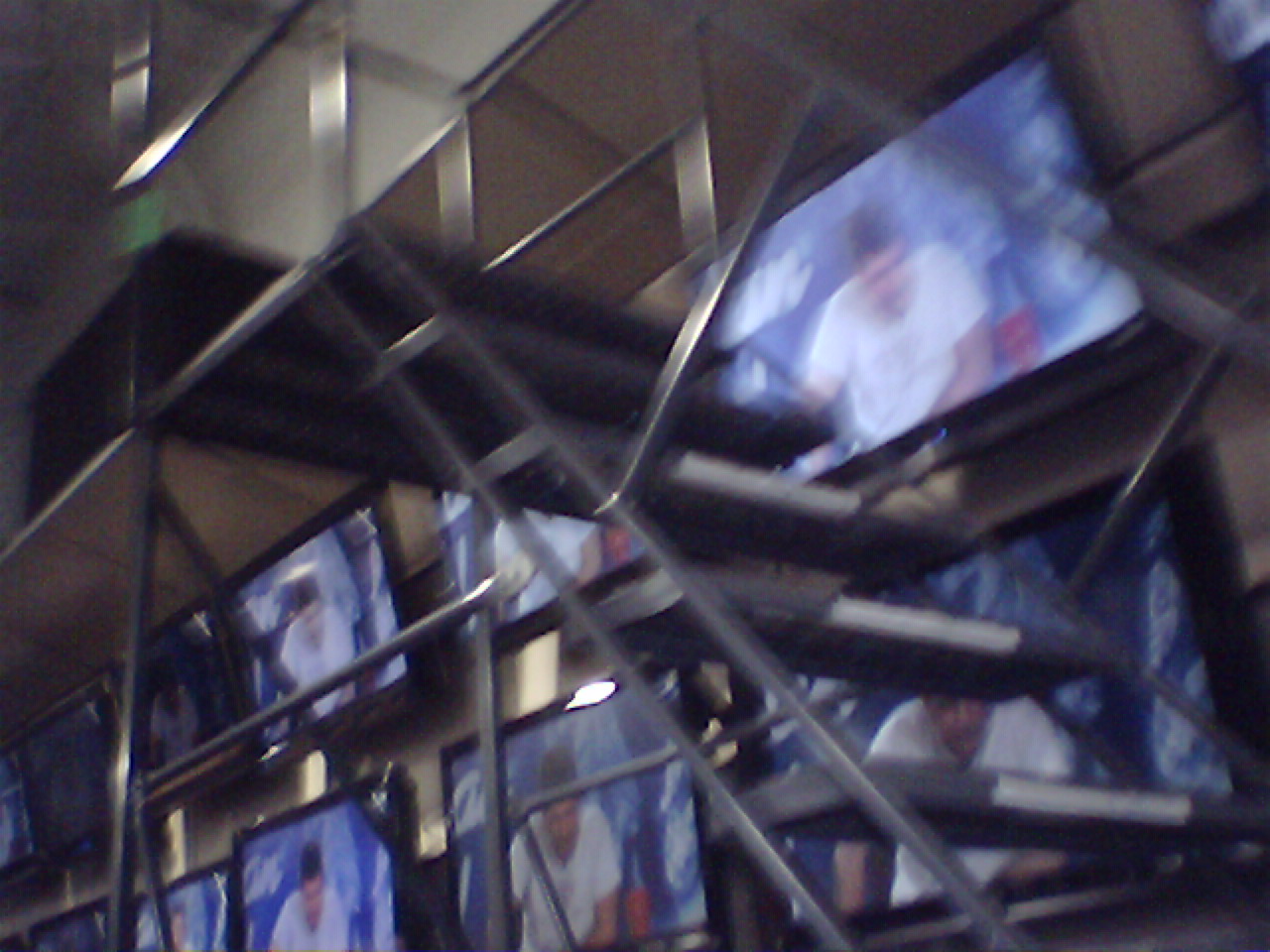The photograph, although slightly blurred, depicts a scene that appears to be inside an electronics store, reminiscent of places like Best Buy. The primary focus is a wall covered with multiple television screens, all showing the same image. The screens display a man with short dark hair and light skin, wearing a white t-shirt, set against a blue background. There seems to be some indiscernible blurred writing near his left side. The TVs, each with a black frame, are arranged in two rows stretching across the width of the photograph.

A metallic frame surrounds the wall, and there's a steel staircase or scaffolding in front of the TV displays, leading upwards with a stair rail. The stairs and scaffolding are composed of gray and silver metal. Above the screens, the ceiling appears dark brown, transitioning to a tan color, with a greyish patch at the top left corner. Notably, there's a slight green splodge just under the metal staircase at the top left. The overall composition suggests an in-store display of televisions, possibly intended to showcase their visual capabilities.